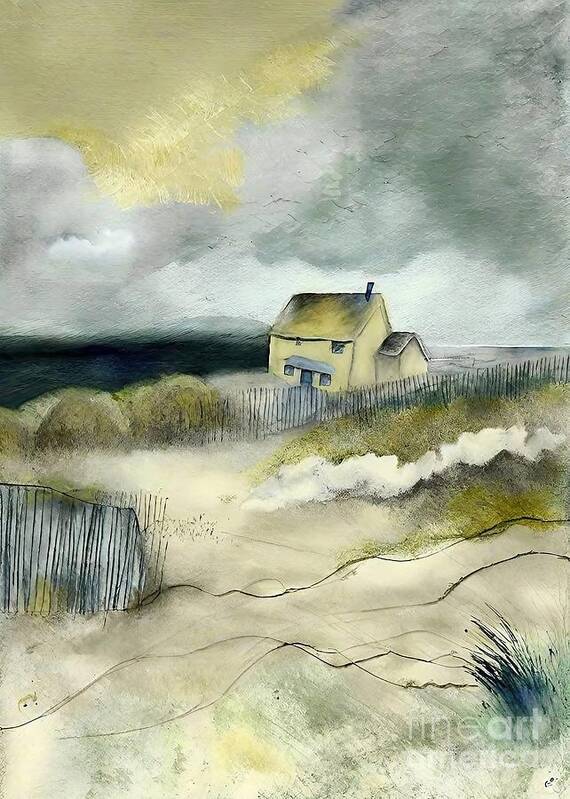The painting depicts a small, tan, two-story house situated on a secluded beach. The house is surrounded by a grayish fence, with another disjointed section of fencing visible in the bottom left of the image. Small bushes dot the sandy, hilly terrain, which is not quite dune-like. In the bottom right, a scrubby plant distinct from the bushes is noticeable. The sky is a complex mix of light and dark gray storm clouds, with a streak of golden sunlight breaking through the top left, creating an almost abstract effect. In the background center left, the dark expanse suggests a vast ocean or sea. The overall painting has an unrefined, almost crude quality, with elements that appear roughly constructed, adding an abstract, expressive touch to the scene.